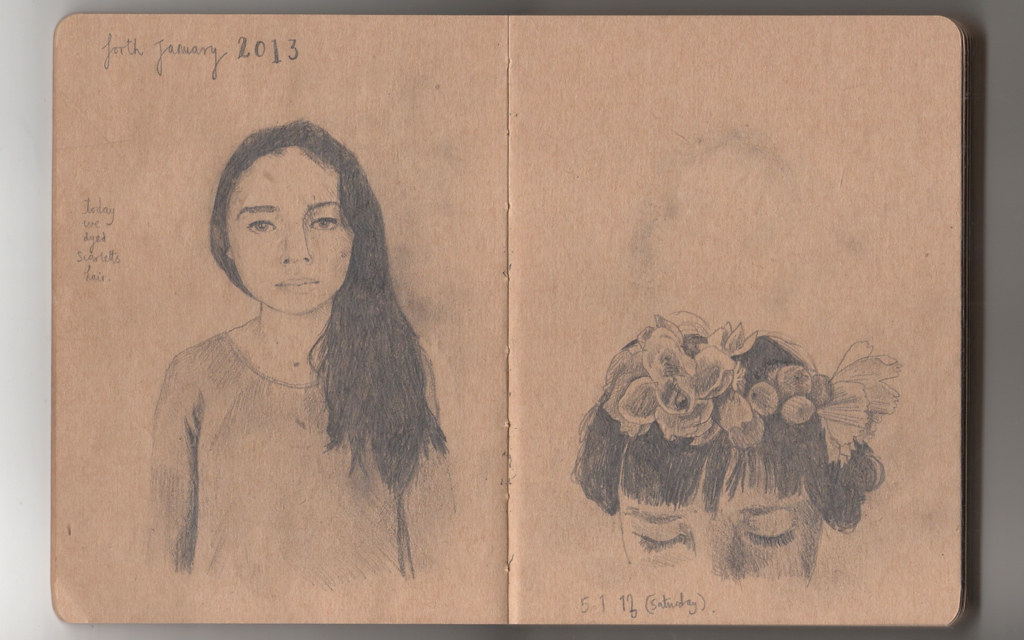The image depicts an open, light brown Moleskine-style journal with two adjacent pages, each featuring a pencil drawing and handwritten text. On the left page, dated "4th of January 2013," is a finely detailed sketch of a young woman with long black hair draped over one shoulder, wearing a simple brown shirt. Above the drawing, the text reads "Today we dyed Scarlett's hair." The woman is looking directly at the viewer with dark eyes and eyebrows, exuding a youthful, pretty appearance.

The right page, dated "5th January 2013, Saturday," contains another pencil sketch of a woman with short hair just above her ears and adorned with flowers. This young woman has her eyes closed, showcasing long dark lashes and bangs. The setting background of both pages is gray, and the booklet itself resembles a small, old-fashioned passport with a brown border.